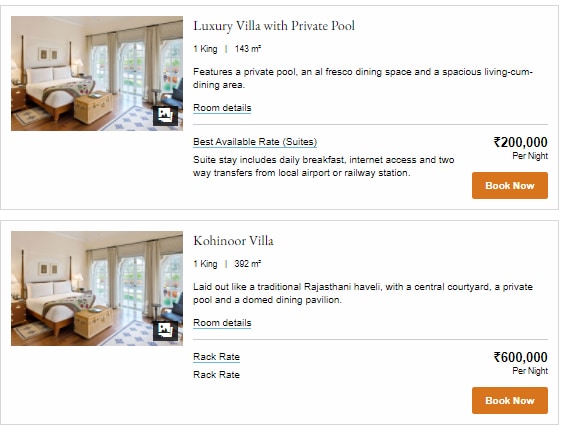This image is a horizontally rectangular screen grab from a travel website, showcasing two luxury accommodation listings. The first listing is for a "Luxury Villa with Private Pool," offering a suite with one King bed and spanning 143 square meters. The villa boasts a private pool, alfresco dining space, and a spacious living-cum-dining area. Room details linked via a blue line include the best available rate, daily breakfast, internet access, and two-way transfers from the local airport or railway station. The cost is $200,000 per night, with a prominent "Book Now" button available.

The second listing is for the "Koh-i-Noor Villa," also featuring a suite with one King bed but covering a more expansive 392 square meters. This villa is designed in the style of a traditional Rajasthani Haveli, complete with a central courtyard, private pool, and domed dining pavilion. The nightly rate for the Koh-i-Noor Villa is $600,000, and it also includes a "Book Now" button.

Interestingly, the same image is used for both listings despite the significant differences in price and location.